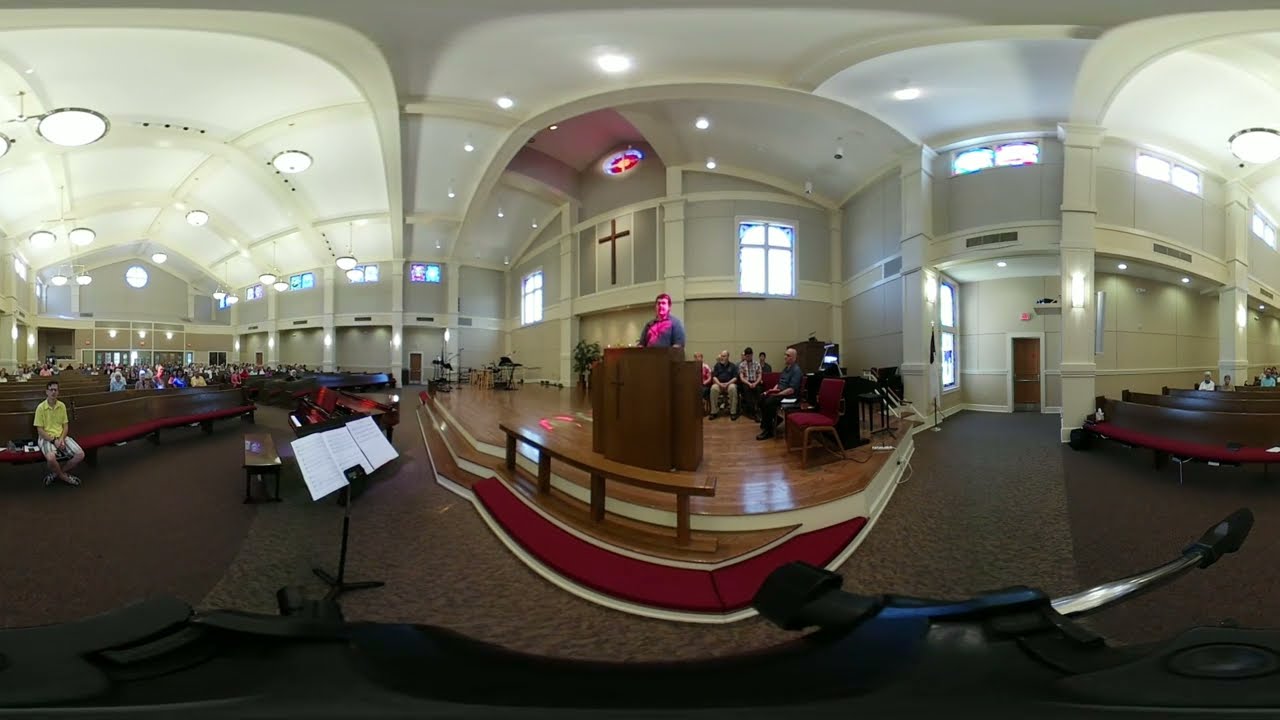This photograph captures the interior of a church taken with a fisheye lens, producing a distorted perspective. Dominating the center of the image is a hardwood stage with a man standing behind a podium, presumably delivering a speech or sermon. At the lower front part of the image, there is a music stand and what appears to be a warped microphone. The floor is carpeted in gray with a red runner leading to the altar. A cross is prominently displayed above the podium, and a striking stained glass window adorns the upper part of the wall behind the altar. To the left of the stage, several benches accommodate sparse parishioners, most sitting towards the back, except for one individual in yellow and gray-striped shorts seated in the front row. Additional details include various colored elements such as brown, black, white, yellow, red, blue, purple, and tan, contributing to the rich visual tapestry of the church's interior.